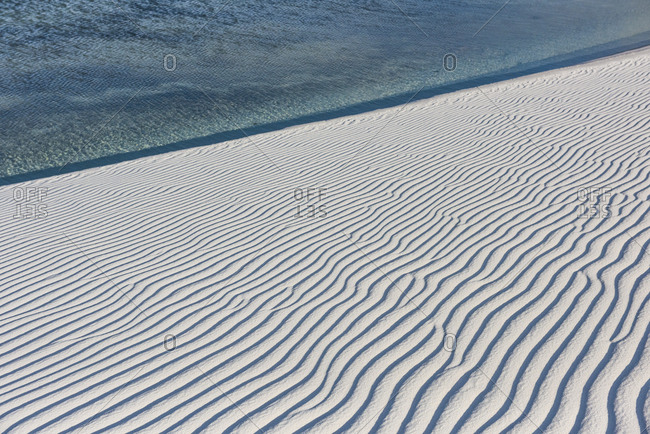The rectangular image, slightly wider than it is tall, captures a serene coastal scene. On the right side, there's a pristine beach with white sand. The sand features wavy, evenly spaced lines running from left to right, intersecting and creating a rippled effect. This pattern leads down to the water's edge, located on the left side of the image. The water, with its clear blue hue, transitions from a darker shade near the shore to a lighter blue further out, where faint dark specks are visible on the top left. The image is overlaid with faint gray watermark lines forming a diamond grid, with intersecting points marked by zeros and the word "offset." The letters "OFF" are properly oriented, while "SET" is upside down. A blue stripe diagonally cuts across the picture, slightly above the halfway mark from the left bottom corner to near the upper right corner. Above this line, the color seamlessly blends into a predominantly blue shade with hints of sand color below. The combination of these elements creates a visually striking image, enhanced by the intricate overlay of text and lines.